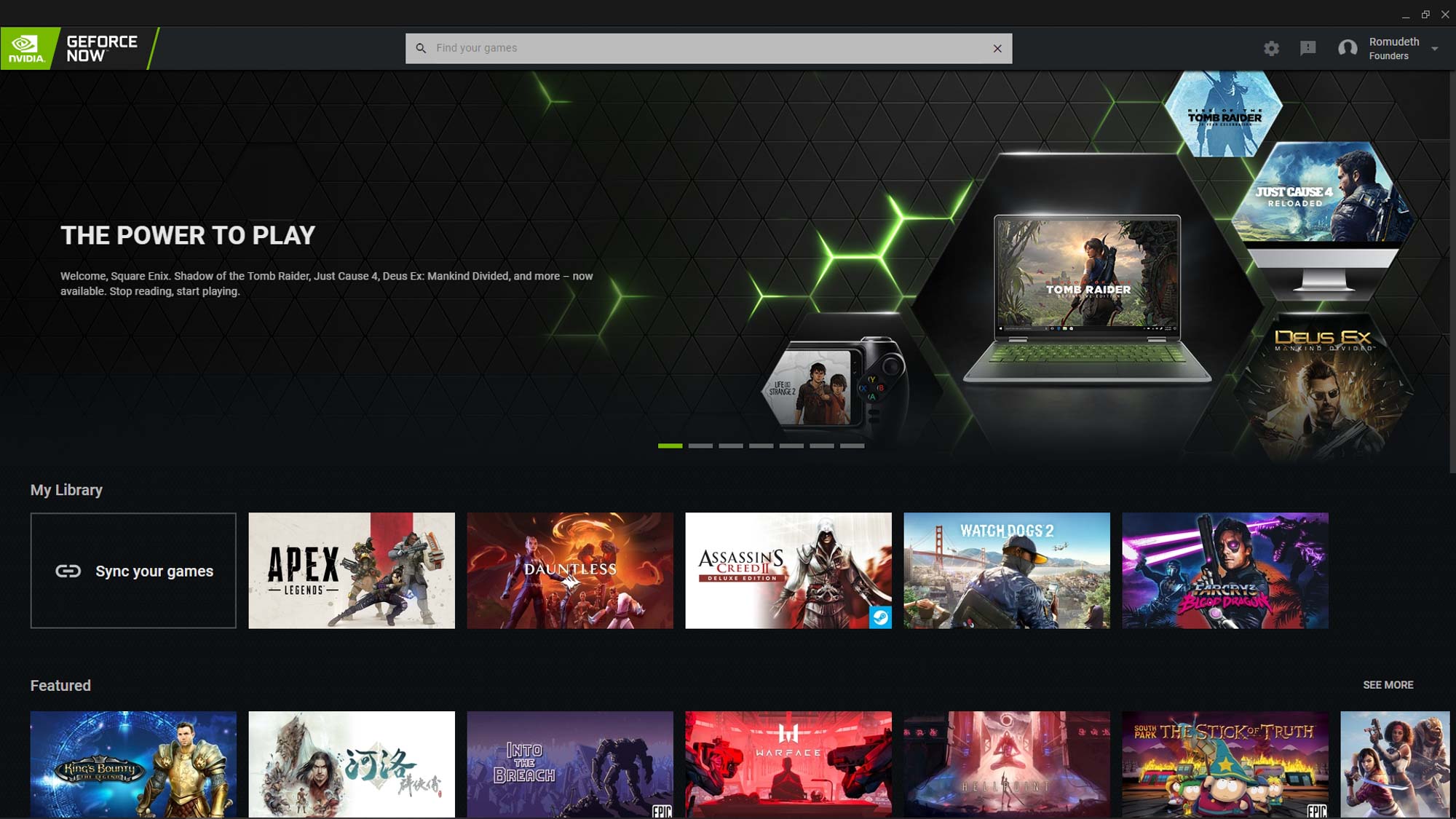Here's a cleaned-up and detailed caption for the image:

---

The screenshot captures the homepage of the G4Snail website, characterized by a predominantly black color scheme with striking neon green accents. The top half of the screen features a honeycomb pattern outlined in neon green, reminiscent of a beehive. This section highlights a computer nestled within one of the honeycombs and displays various video games including "Tomb Raider." Below the honeycomb, an extensive list of 18 video games is presented, with notable titles such as "Apex Legends," "Dauntless," "Assassin's Creed," and "Watch Dogs 2." The games are organized into categories like "My Library" and "Featured," the latter showcasing five highlighted games. The sleek design combines hexagonal shapes and vibrant neon elements, creating a visually engaging interface for gamers.